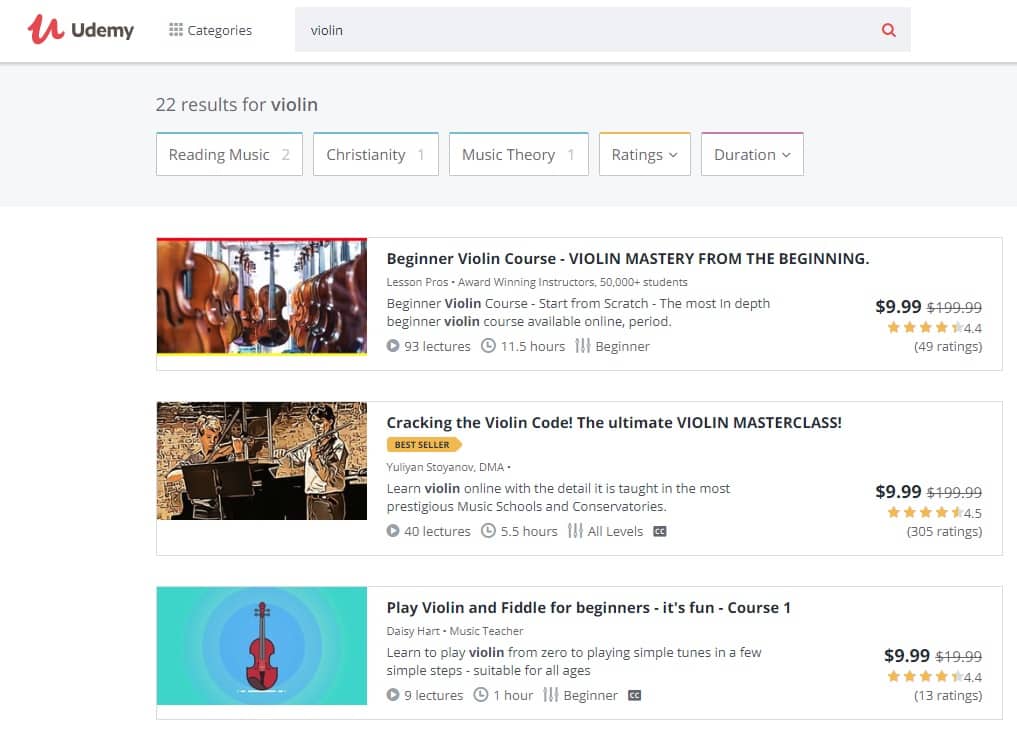**Website Screenshot Description: Udemy Search Results for Violin**

At the top left corner of the website, there is a red "U" logo followed by the word "Udemy." Adjacent to "Udemy," there is a grid icon labeled "Categories." A search bar displays the word "violin," accompanied by a red magnifying glass icon. Below the search bar, it indicates that there are "22 results for violin," broken down into subcategories: "Reading Music (2)," "Christianity (1)," and "Music Theory (1)."

Sorting options labeled "Ratings" and "Duration" each feature a down arrow for further refinement of search results. 

A prominently displayed image depicts around 15 violins brightly lit. The featured course titled "Beginner Violin Course: Violin Mastery from the Beginning" is presented by "Lesson Pros, Award-Winning Instructors," boasting "50,000 students." This course is described as "the most in-depth beginner violin course available online," with a runtime of "11.5 hours." It is priced at "$9.99," discounted from "$199."

Another course listed is "Cracking the Violin Code: The Ultimate Violin Master Class," which offers detailed instruction taught at some of the most prestigious music schools and conservatories. This course, also priced at "$9.99," features images of a couple of people playing the violin.